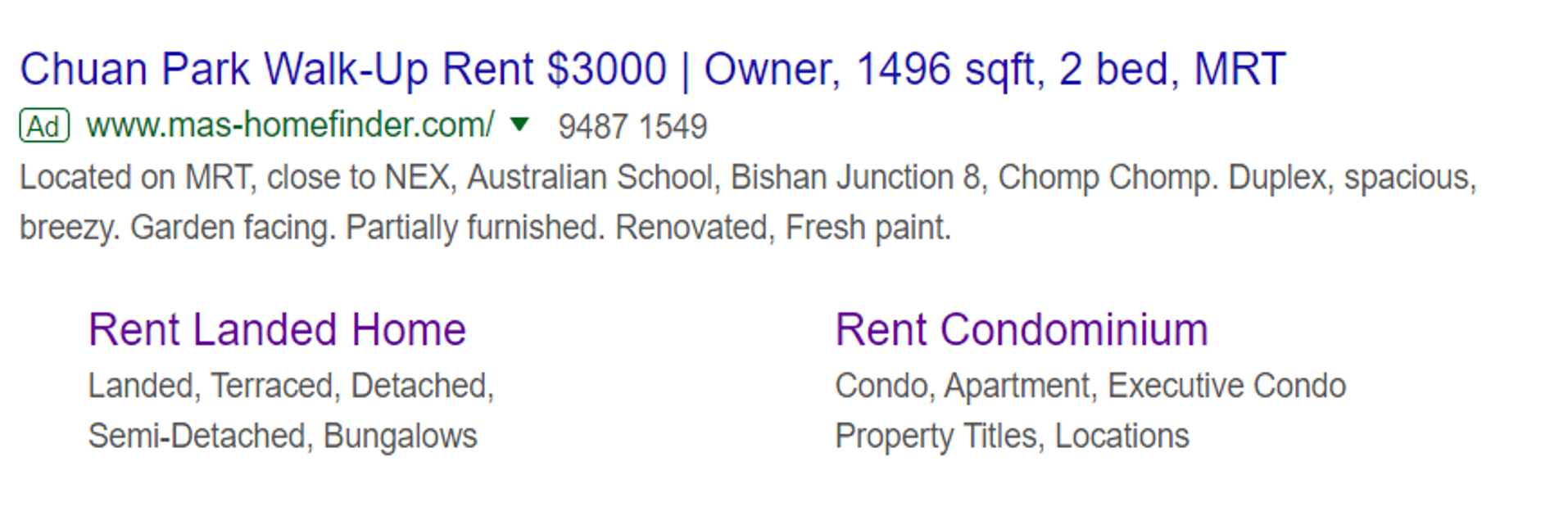The image is an advertisement on a white background featuring detailed property information. At the top left, written in blue text, the ad reads: "Chwan Park Walk-Up, Rent $3,000, Owner, 1496 sq. ft., 2-Bed, MRT." Below, in green, the ad includes a website link: "www.mashomefinder.com/94871549."

Going from left to right, the ad highlights various nearby amenities and features, including proximity to the MRT, NEX, Australian School, Bishan Junction 8, and Chomp Chomp. The property is described as a duplex that is spacious, breezy, garden-facing, partially furnished, and recently renovated with fresh paint.

To the left of the ad, there is a section that lists different types of landed homes available for rent, which include: "Landed, Terraced, Detached, Semi-Detached, Bungalows." 

On the right side, there is a similar section for condominiums, which lists: "Condo, Apartment, Executive Condo, Property Titles, Locations."

The sections "Rent Landed Home" and "Rent Condominium" are highlighted in purple, indicating they are clickable links.